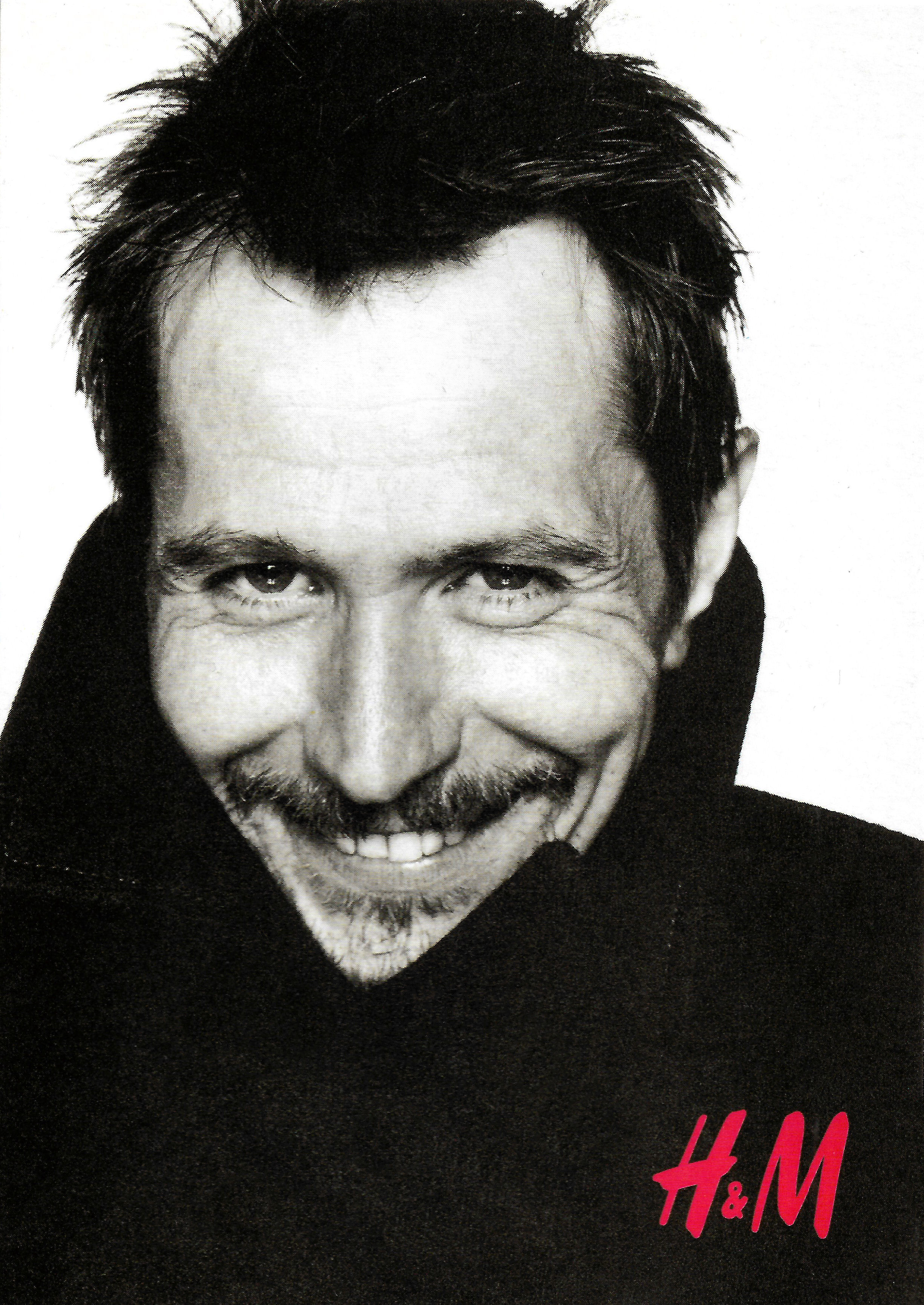This black and white promotional photo for H&M prominently features actor Gary Oldman in a striking close-up. Oldman, slightly left of center in the image, exudes charisma with a mischievous grin that reveals his teeth. His medium-length dark hair, complete with a widow's peak, adds to his enigmatic presence. He sports a five o'clock shadow beard and a small mustache, while his dark jacket—likely a hoodie—features a large collar pulled up around his neck, partially covering his right ear and cheek, but leaving his left ear visible. The high collar outlines his face, adding a dramatic flair to the composition. His eyebrows are slightly lowered, giving one eye a narrower appearance, enhancing his playful and engaging look. Completing the advertisement, the H&M logo stands out in large red letters at the bottom right corner of the image.